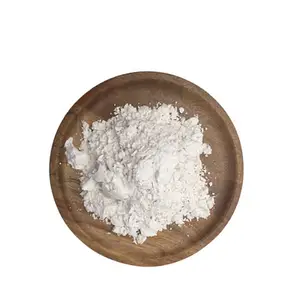In this simple and elegant photo taken from a top-down perspective, a wooden plate with curved edges, crafted in light browns and tans, showcases its intricate wood grain texture. Set against a completely white background that provides no context or distractions, the plate holds a generous pile of finely clumped white powder in its center. The powder, possibly flour, sugar, or salt, creates a beautiful, cloudy, and feathery texture, suggestive of preparation for a baking project. The powder is predominantly centered and mounded high, though small remnants scatter around the indent of the plate, emphasizing its use. The photograph captures the essence of the scene with a stark simplicity and a sophisticated viewpoint, as if taken from a higher angle to fully document the arrangement for a cookbook or similar project.